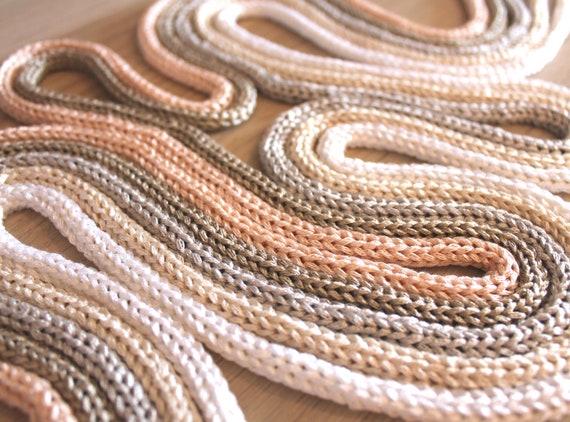The photograph captures a mesmerizing array of thick, crocheted yarns laid out on a wood grain table. These yarns, resembling a snake-like, coiled pattern, stretch and curve in a rhythmic sequence from the bottom left to the top right of the image. Each yarn strand is thick, comparable to a shoestring, and intricately designed, with some appearing almost chain-like. The colors transition fluidly from peach-copper, to khaki, to shades of gray, beige, and finally to white, creating a beautiful gradient across the composition. The yarns are meticulously arranged side by side, maintaining their specific order as they form arcs and deep curves, with some sections positioned closer together. The central darker strand, which stands out most sharply in focus, anchors the image amidst a muted palette and a softly lit setting. As the yarns weave their way through the photograph, parts of the wood table peek through the gaps, adding a textured background to this elegantly detailed, serpentine display.